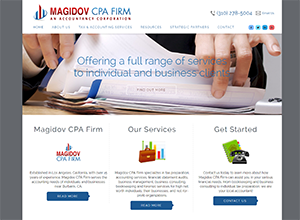This small image appears to be a promotional banner for the Magidov CPA Firm. In the top left corner, there's a bar graph featuring three bars: a blue bar, a red bar, and a green bar, with the red bar significantly taller than the others. Adjacent to this graph, "MAGIDOV CPA FIRM" is prominently displayed, with "MAGIDOV" in red and "CPA FIRM" in blue, both in uppercase lettering. Directly below, there is some red text that is blurry and difficult to decipher. 

On the top right, a gray phone icon is visible, accompanied by a contact number in blue text. Below the phone number are several tabs labeled in blue text which are too small to be read clearly. To the right of these tabs, there are four buttons, each in a different shade: light blue, neon blue, darker blue, and red.

The central portion of the image features an individual flipping through papers, beside which is the text "Offering a full range of services to individual business clients," written in blue. Below this image are three vertically separated columns labeled "MAGIDOV CPA FIRM," "OUR SERVICES," and "GET STARTED." Each column is delineated by a light gray vertical line and contains an image followed by black text comprising several sentences describing the respective section. At the bottom of each column, there is a blue, battery-shaped button pointing to the right, with white text beneath each paragraph.